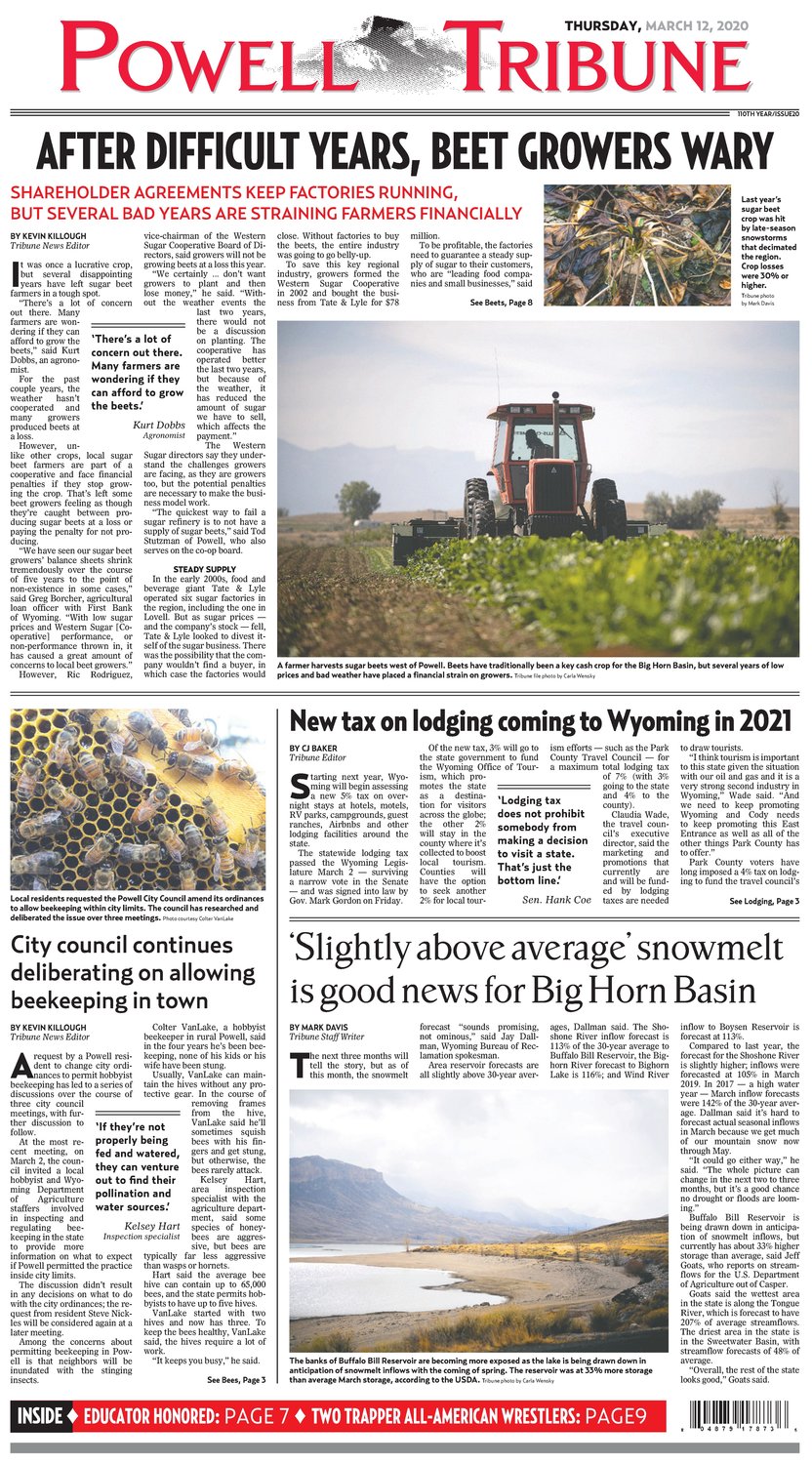This is a vertical image of a newspaper, specifically the front page of the "Powell Tribune," dated Thursday, March 12th, 2020. The header at the top includes "Powell Tribune" in large red letters, accompanied by "110th Year, Issue 20" in black. The header also includes the date and a number of small separating lines for visual structure.

The primary article is headlined in dark, bold, uppercase letters: "After Difficult Years, Beet Growers Weary." A subheading in red adds detail: "Shareholder agreements keep factories running, but several bad years are straining farmers financially." The article is written by Kevin Killough, the Tribune's news editor. Below this, there are pictures, including one of a tractor in a field during harvest, and another showing the sugar beet crop from the previous year.

To the side, another article is titled "New Tax on Lodging Coming to Wyoming in 2021," authored by CJ Baker. Nearby, an article discussing City Council deliberations about allowing beekeeping in town is illustrated with a picture of numerous bees. Additionally, there is an article titled "Slightly Above Average Snowmelt is Good for the Bighorn Basin," written by Mark Davis.

The barcode is visible at the bottom right corner of the page against a white background that seems to blend with the computer screen behind it, creating an illusion of the newspaper seamlessly floating.